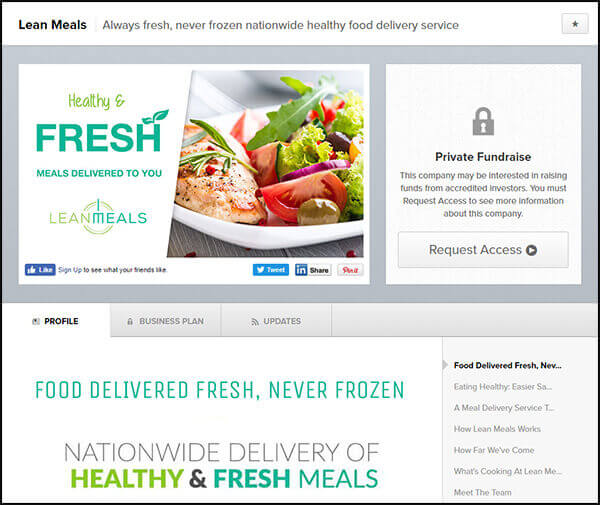![Lean Meals Website Screenshot]

The image showcases a section of the Lean Meals website, a nationwide healthy food delivery service known for its slogan, "Always fresh, never frozen." On the left, the company's branding and tagline are prominently displayed. Below, a white rectangular box set against a gray background contains key social media engagement prompts: "Healthy and fresh meals delivered to you. Lean Meals." accompanied by icons for Facebook (with a prompt to "Like" the page), Twitter (with a share option), and another red icon of unknown purpose. Also featured within this section is an appetizing image of a fresh salad paired with a piece of baked, skinless chicken.

Further down, another white box is dedicated to a "Private Fundraiser," informing visitors that Lean Meals is seeking fundraising from accredited investors and offering a button to request access to more information.

At the bottom, three tabs provide navigational options. Two gray tabs labeled "Business Plan" and "Updates," and a white tab labeled "Profile." Below this section, text reiterates the company's mission of "Food delivered fresh, never frozen, nationwide delivery of healthy and fresh meals." On the right side, a partially visible snippet emphasizes the ease of eating healthy with Lean Meals: "Food delivered, never...NEV...eating healthy, easier...SA...a meal delivery service...T..."

The combined elements paint a clear picture of Lean Meals as a convenient, health-focused meal delivery service actively seeking investment to expand and improve its offerings.